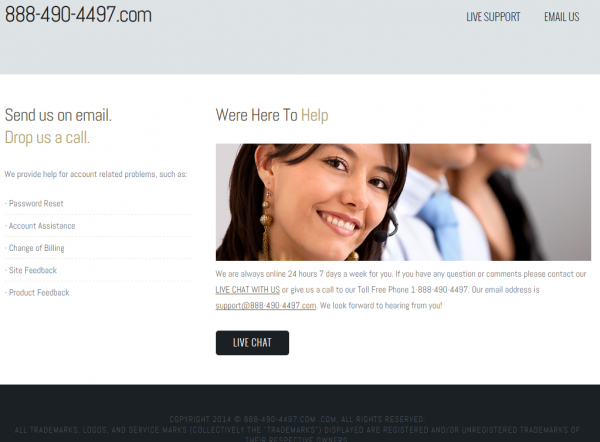This image is a screenshot of a website featuring a horizontally elongated layout. At the top, there is a light gray header with bold black text in the upper left corner showing a combined phone number and website URL: "888-490-4497.com". On the upper right corner of the header, the options "Live Support" and "Email Us" are displayed.

Beneath the header, the main area of the webpage features a white background. Centrally displayed is a color photograph of an attractive young woman. She has dark eyes, dark hair, and is adorned with gold earrings. Her smile is welcoming and engaging. Flanking her are two individuals, though only the front of their chests and chins are visible.

Above the young woman's head, in brown text, it says, "We're here to help." Below her image, there's an informative message: "We are always online, 24 hours a day, 7 days a week for you. If you have any questions or comments, please contact our live chat via the 'Chat with Us' link or call our toll-free number: 1-888-490-4497."